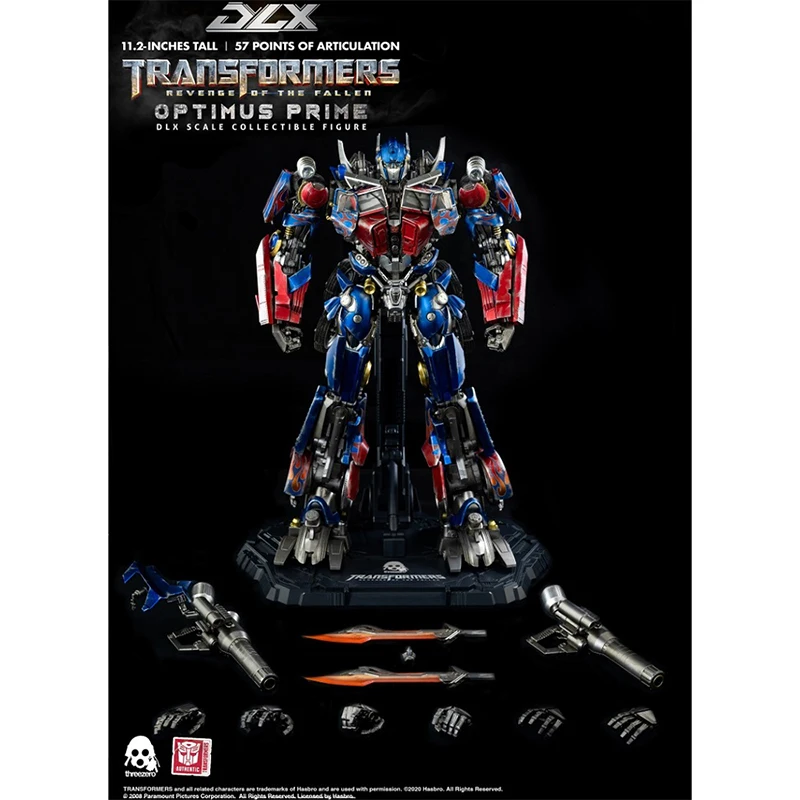The advertisement poster features a meticulously detailed image of a DLX Transformers Optimus Prime collectible figure, prominently set against a stark black background. Standing at 11.2 inches tall with 57 points of articulation, the meticulously crafted figure showcases Optimus Prime in vivid red, blue, and silver colors, with a touch of gray, perched on a dark gray podium. Surrounding the iconic Transformer are an array of interchangeable accessories, including two intricately designed guns, two swords with gray and red accents, and six variations of hands for dynamic posing possibilities. The upper left corner of the poster highlights essential text in white and silver, stating "DLX Transformers Optimus Prime: A DLX Scale Collectible Figure" along with other attributes. The bottom left corner features the transformative logos and manufacturer logos, adding an official seal to this highly detailed collector's item.